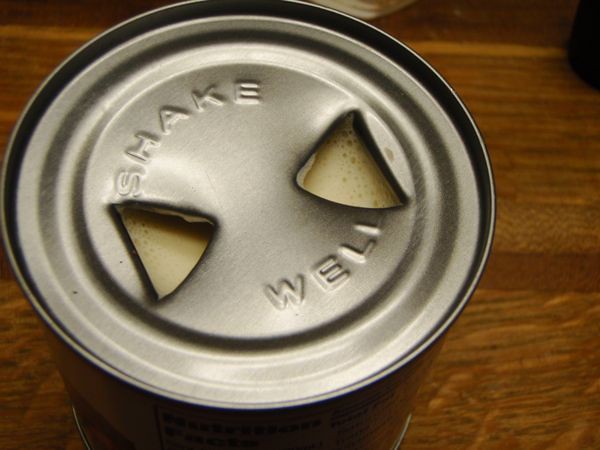This image depicts the top of a round aluminum can, placed on a brown, lined table. The silver top is embossed with the words "shake well," with "shake" arcing along the upper edge and "well" along the lower edge of the circular top. In the center between these inscriptions, there are two triangular openings, their bases towards the outer edge and tips pointing inward towards each other. Through these openings, a bubbly, creamy substance is visible, hinting at the can’s contents. The surface around the opening triangles appears to have a goldish, copperish, grayish hue, adding a slight color variation to the otherwise silver top. The wrapped sides of the can exhibit an orange and yellow color scheme.